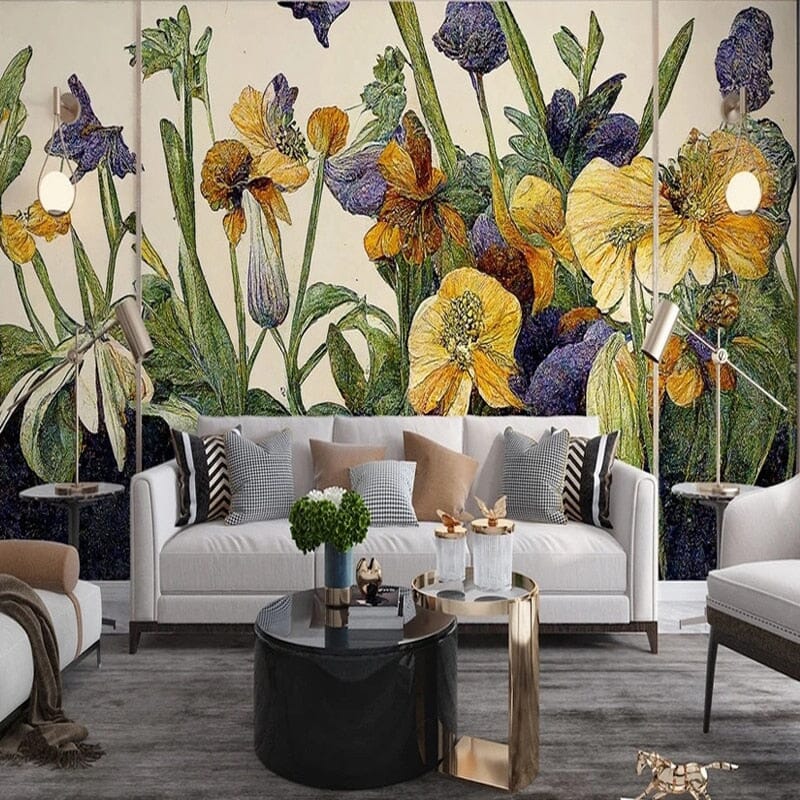The photograph showcases a contemporary living room designed by an interior designer. The focal point of the room is the stunning back wall adorned with a large-scale floral mural featuring grand flowers in shades of purple, gold, and yellow with green stems and leaves. This mural is set against a cream or off-white background, creating an impressive graphic feature. 

In front of this mural, a modern white sofa with brown legs is prominently displayed, accented by checkered and solid colored pillows in shades of brown, gray, and black. To the left of the sofa is a matching white chaise lounge with a brown cylindrical pillow and a dark brown throw draped across it. To the right is a white armchair, completing the seating arrangement.

A circular black lacquer coffee table with a marble or glass top sits centrally in front of the sofa. This table features a vase of greenery and white flowers, a blue vase with a silver base, and a gold fish sculpture. Attached to this coffee table is a smaller gold circular table with a square base and a glass inset tabletop, holding two glass jars with butterfly lids. Additionally, two small end tables flank the sofa, each with a white top and a brown base.

The floor consists of planking designed to resemble old, restored barn wood, adding a touch of rustic charm to the contemporary space.